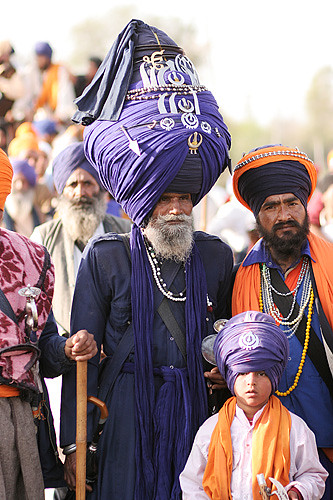The photograph depicts a group of Sikh men and a young boy, all adorned with colorful turbans and scarves, emphasizing a rich cultural and religious setting. In the foreground, five individuals stand out clearly. On the left, a person is partially visible, wearing a pink and red shirt, holding a walking stick. Next to him, a man with a majestic, tall purple turban, complemented by a blue long-sleeved shirt and a purple scarf, steps forward. Beside him is another man in an orange turban, blue shirt, and an orange scarf around his neck.

A young boy stands in front of them, wearing a white shirt, an orange scarf, and a purple turban adorned with a prominent symbol. Another figure in the background features an older man with a long, white beard and a blue turban, dressed in a white and grey robe. The background is blurred, revealing only the faint outlines of additional people, suggesting a gathering or religious ceremony.

The central figure is notable for his large blue turban decorated with beads and gold pins, a grey beard and mustache, and a blue scarf. He appears dignified, with a curved knife at his side, reflecting the attire and symbolism often associated with Sikh ceremonies. The vivid descriptions and specific details provide a cohesive and richly detailed portrayal of the scene.